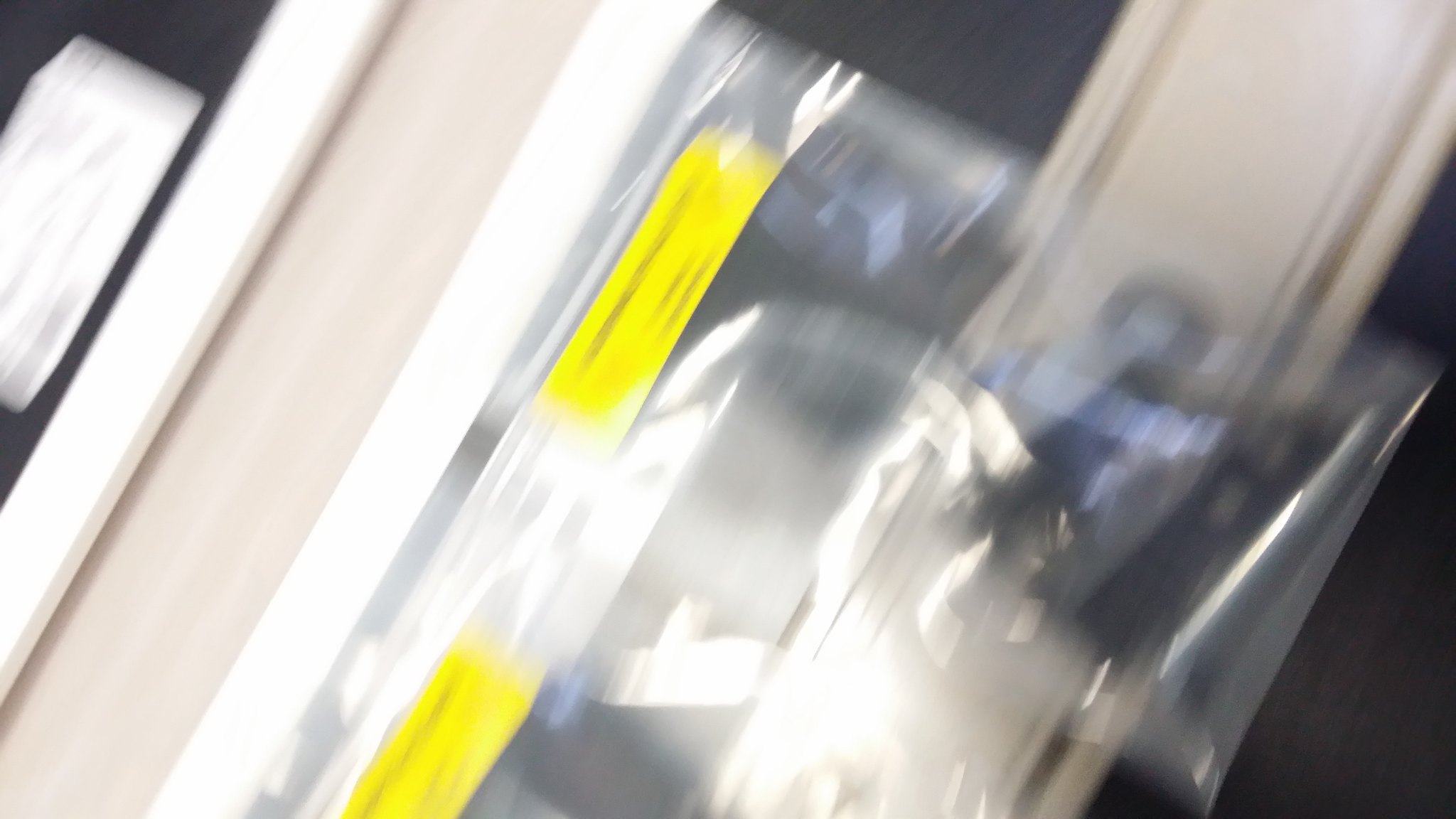The image is very blurry and difficult to decipher, likely taken in motion. It appears to depict a beige-colored wall or surface with white trim or molding, partially obscured by a large clear plastic wrap material. The plastic, positioned centrally, features two yellow rectangular stickers or labels with unreadable black text. The scene suggests additional elements, such as a possible black hanger within the plastic. To the sides of the plastic, there are black sections that might indicate paint or the frame of a doorway. The overall perspective is tilted, as if the entire setup is at an angle. Additionally, in the top left corner, there's a small white labeling paper with illegible writing. Some beige protrusion extends from the far right side of the plastic, adding to the image's complexity.